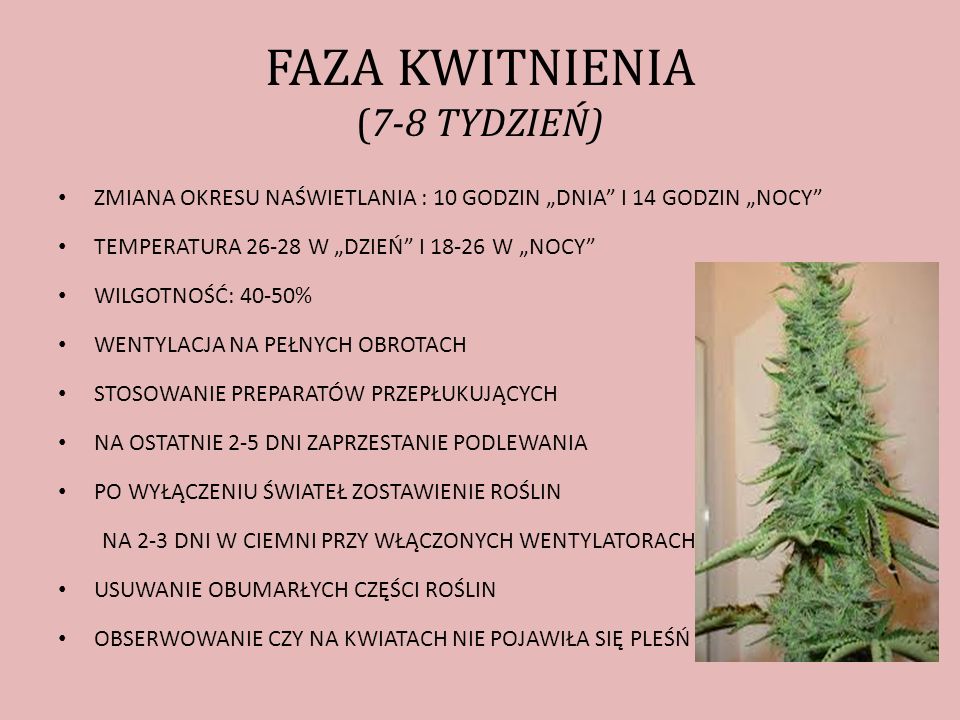The image portrays a pink background, possibly a slide from a presentation, featuring black text in all capital letters which appears to be in Polish. At the top of the slide, a title reads "FASA QUINTINENDA," followed by italicized text in parentheses that reads "(7-8 TIZIAN)." Below this, there are nine bullet points represented by dark black circles. To the right of the text, there is a photograph of a green plant or tree with long, spiky leaves, resembling a pine tree, standing against a dull peach-colored wall. A section of a door or window can be seen beside the plant, where light from outside creates shadows along the borders. The text on the slide provides instructions related to plants, advising to leave them in a dark room with fans on for two to three days, remove dead parts, and observe for mold on the flowers.